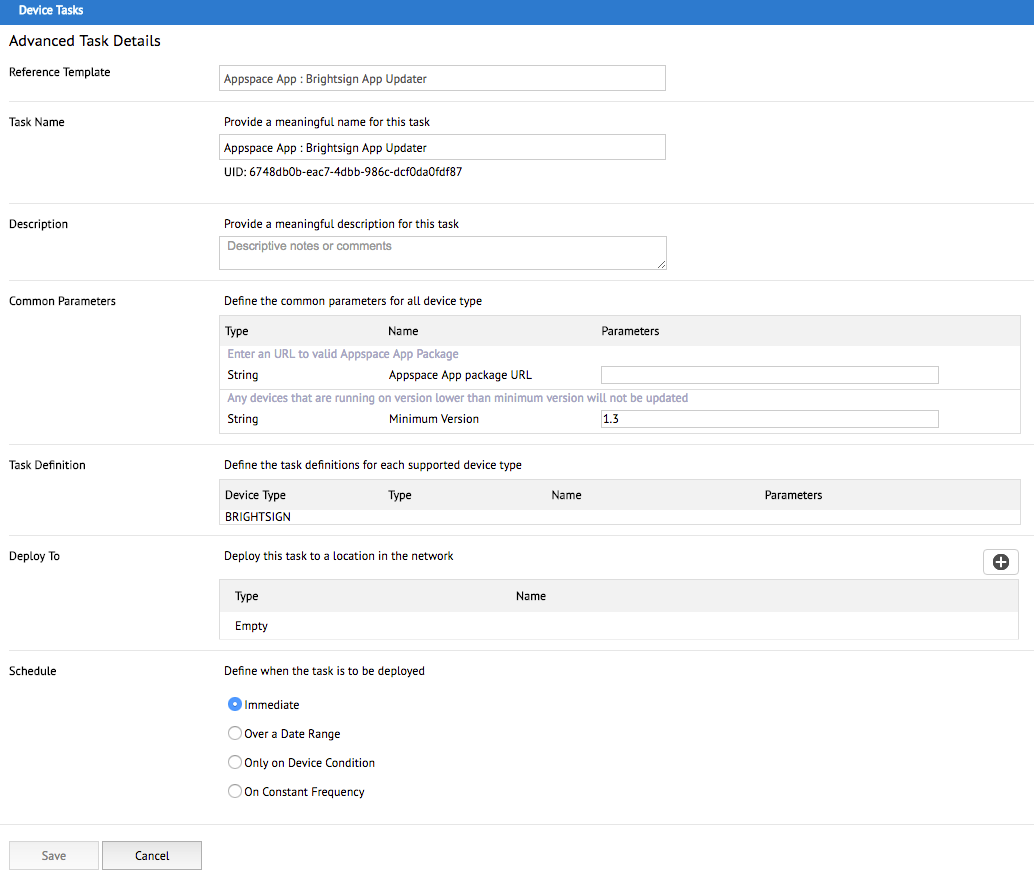The image features a user interface with a clean, white background. At the top, a slim blue banner spans the width of the image, containing white text in the upper left corner that reads "Device Tasks." Below this banner is a structured layout of sections and input fields for detailed task configuration.

The "Advanced Task Details" section is followed by a "Reference Template" heading. Below these, a text box labeled "AppSpace App, BrightSign App Updater" is displayed, containing instructions to "provide a meaningful name for this task" and suggests the name "AppSpace App: BrightSign App Updater," along with a unique identifier (UID) number underneath.

In the "Description" section, users are prompted to "provide a meaningful description for this task," with a box available for entering additional descriptive notes or comments.

The "Common Parameters" section allows users to "define the common parameters for all device types," including a field to "enter a URL to a valid AppSpace app package."

Next, in the "Task Definition" section, users can "define each task for each supported device type." For the "Device Type" field, "BrightSign" is indicated. The "Deploy To" field prompts users to specify a location in the network, and the type is currently marked as "empty."

The "Schedule" section offers various deployment timing options: "Immediate," "Over a Date Range," "Only on Device Condition," and "On Constant Frequency," with "Immediate" being pre-selected.

At the bottom left corner of the interface, there are two buttons: one for "Save" and one for "Cancel."